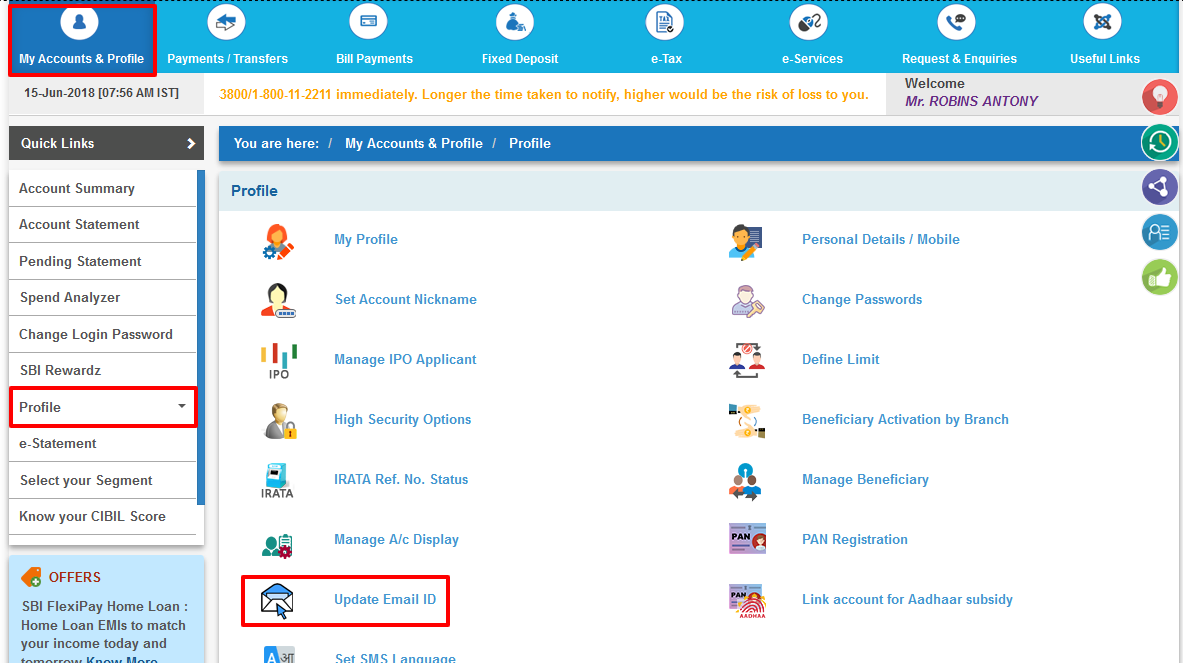This web page is bustling with various features and options, giving it a complex layout. At the very top, a blue navigation bar stretches horizontally across the screen, adorned with a series of icons. The icon at the very left upper corner, outlined in red, is labeled "My Accounts and Profile." Following it in sequence are other icons labeled Payments, Transfers, Bill Payments, Fixed Deposit, eTax, eServices, Requests and Inquiries, and Useful Links.

In the main section of the page, the user's Profile is prominently displayed. This section, titled Profile Info, is populated with numerous colorful, stock photo-esque icons. These icons depict simple cartoon figures, stripped of facial features, and each one represents different settings that the user can manage. These settings are organized into two columns and include options such as My Profile, Set Account Nickname, Manage IPO Applicant, and High Security Options.

On the left side of the page, a vertical menu labeled Quick Links provides additional navigation options including Account Summary, Account Statement, Pending Statement, Spend Analyzer, among others. Notably, the Profile section within this vertical menu is outlined in red, drawing attention particularly to the Update Email ID option, which is also highlighted with a red outline.

Finally, in the upper right corner of the screen, there are five small circular icons, likely functioning as share buttons and like buttons, rounding out the interface by offering social media integrations or interactive features.

This detailed layout provides ample navigation and functionality to manage various personal and financial tasks directly from the web page.